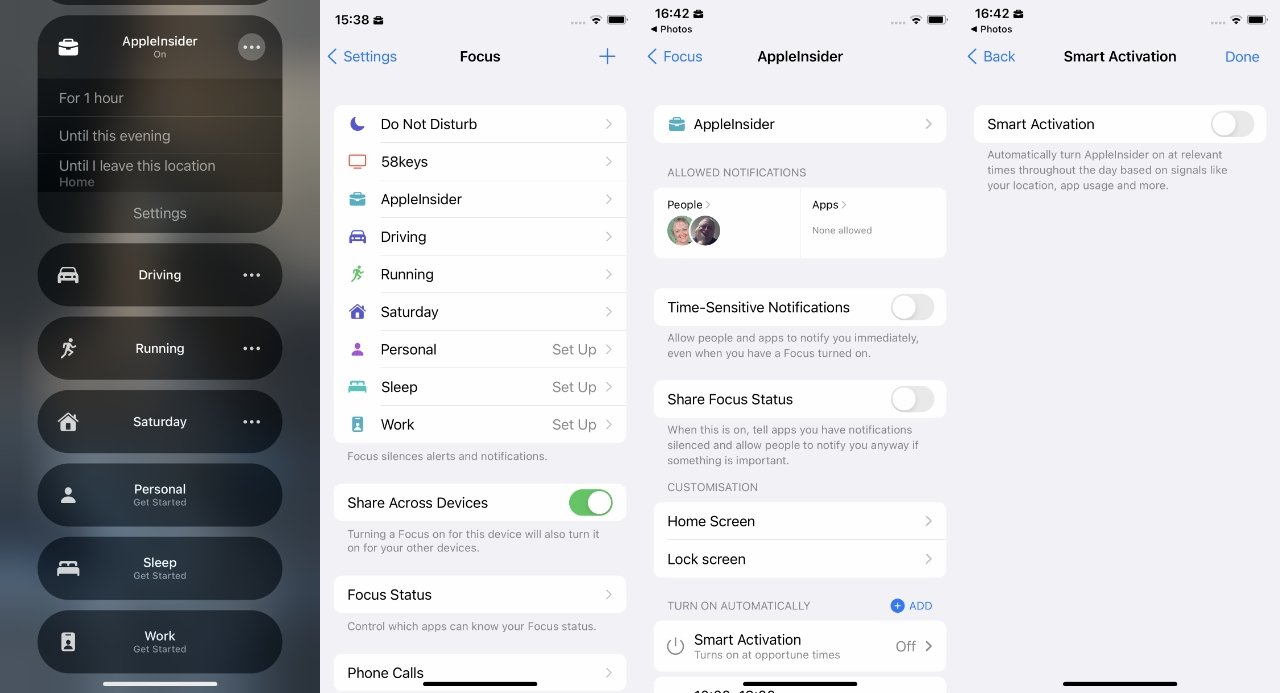Here is a detailed and cleaned-up caption for the described image:

---

The image consists of four screenshots taken from a mobile device, showcasing various "Focus" settings and configurations. 

1. **First Screenshot:** 
   - The screenshot features a gray, opaque background with several widgets in black. 
   - At the top, the largest widget is a square that reads "Apple Insider" in white at the top, followed by options in gray text such as "1 Hour," "Until This Evening," "Until I Leave This Location," and "Home." At the bottom of this square widget, there is a "Settings" option.
   - Below the square widget, there are several smaller, horizontally rectangular widgets:
     - "Driving" with a white car icon on the left and three white dots on the right.
     - "Running" with a white stick figure icon on the left and three dots on the right.
     - "Saturday" with a house icon on the left and three dots on the right.
     - "Personal" with a profile icon on the left and "Get Started" text beneath it.
     - "Sleep," with a bed icon on the left and "Get Started" text underneath.
     - "Work," with a name tag icon on the left and "Get Started" text under it.

2. **Second Screenshot:**
   - This screenshot displays the "Focus" settings page.
   - The top bar shows "Focus" with "Settings" on the left and a "+" sign on the right.
   - Several options are listed within white boxes such as "Do Not Disturb," "58 Keys," "Apple Insider," "Driving," "Running," "Saturday," "Personal," "Sleep," and "Work" with a right-facing caret next to each.
   - For "Personal," "Sleep," and "Work," there is a "Set Up" option with a right-facing caret. 
   - Below these options, the text "Focus silences alerts and notifications" appears.
   - Another white box labeled "Share Across Devices" contains a toggle button in the "On" position, with explanatory text beneath.
   - Additional settings include "Focus Status" and "Phone Calls," each within a white box and with a right-facing caret.

3. **Third Screenshot:**
   - Displaying a specific "Focus" setting labeled "Apple Insider."
   - The top bar shows "Apple Insider" with a back button on the left and a "Focus" title.
   - The main white box at the top has a blue briefcase icon next to "Apple Insider," followed by another caret.
   - Below this, the section labeled "Allowed Notifications" includes:
     - A "People" section with avatars of an older man and woman on the left and an "Apps" section on the right stating "None Allowed."
     - A white box labeled "Time-Sensitive Notifications" with a toggle button that is off. 
     - An explanation that allowing people or apps to notify you immediately even when the focus feature is on.
   - Additional settings include "Share Focus Status" (toggled off), with grey explanatory text, "Customization" options for the home screen and lock screen, and an automatic focus section with a plus sign for adding new setups.
   - A "Smart Activation" setting showing the feature turned off.

4. **Fourth Screenshot:**
   - This shows the "Smart Activation" feature of "Apple Insider."
   - The top bar displays the title "Smart Activation," with a back button on the left and a "Done" button on the right.
   - A white box shows "Smart Activation" being toggled off.
   - Below this, small gray text explains the purpose of this feature, mentioning automatic activation based on signals like location and usage.
   - The remainder of the background is filled with blank gray space.

---